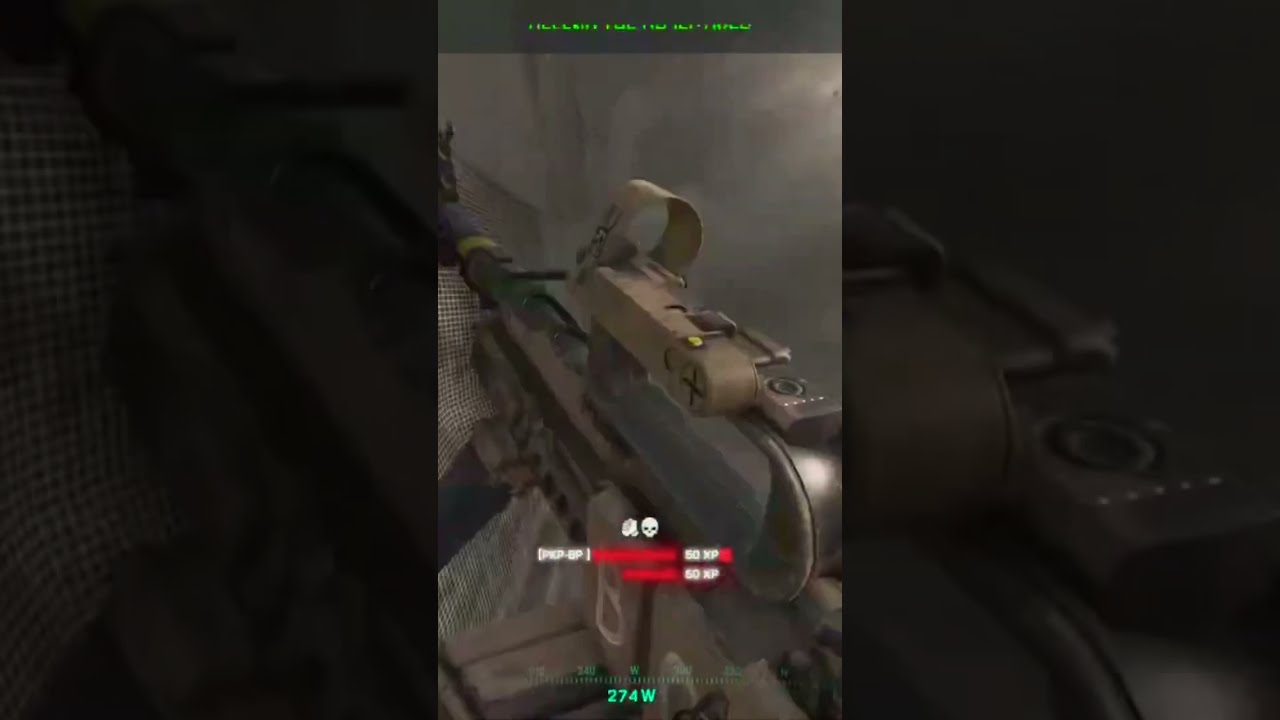This image is a screen capture from a first-person shooter video game, likely adapted for a smartphone or a section of a PC game. The perspective is from the player's viewpoint, showing them holding a gun, possibly an automatic weapon or machine gun with distinct brown and black coloring. The setting appears dark, dominated by grey, brown, and black tones, suggesting a grim, industrial environment, potentially on a walkway, bridge, or in a building with metal grates and smoke. 

At the top of the screen, there is unclear green text. A prominent element is the green directional reading "274W" at the bottom, indicating the player's facing direction. Visible are two red XP progress bars, with "50 XP" labels, one of which is full while the other is half-full. Centrally placed below these bars is a skull icon, likely representing a lifeline or score tally for the player. The overall scene implies an intense and gritty atmosphere within the game.